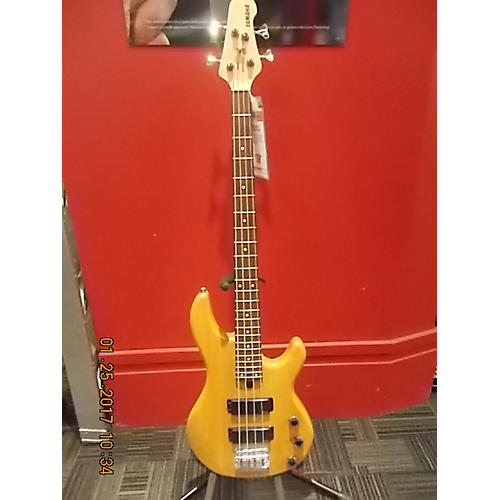In the image, an electric guitar is positioned vertically on a stand against a bright red wall. The guitar has a unique and distinctive shape, with the body being a light brown or yellowish color, the neck a darker brown, and the head a very light natural wood. Its four silver strings run along the fretboard, leading to silver tuning keys at the top. A tag, likely containing a description or price, hangs from the guitar on the right side. Behind the guitar, only the lower edge of a poster is visible. The floor consists of gray carpet squares, suggesting a DIY installation. A date stamp on the left side of the image reads "01/25/2017" with the time noted as "10:34".